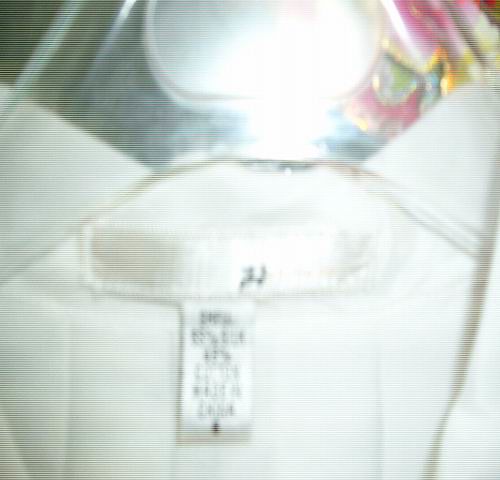The image showcases a sophisticated white blouse elegantly draped on a silver hanger. The garment’s design features a neat, cream-colored rectangular tag stitched inside, near the neckline, highlighting a minimalist elegance. Attached to this primary tag is a secondary care label providing detailed instructions on washing, heat settings, and fabric composition, ensuring proper maintenance of the blouse. The care label also includes essential information such as the blouse's size and material, whether it is made of polyester, cotton, or a blend, ensuring the wearer can keep this refined garment in pristine condition.